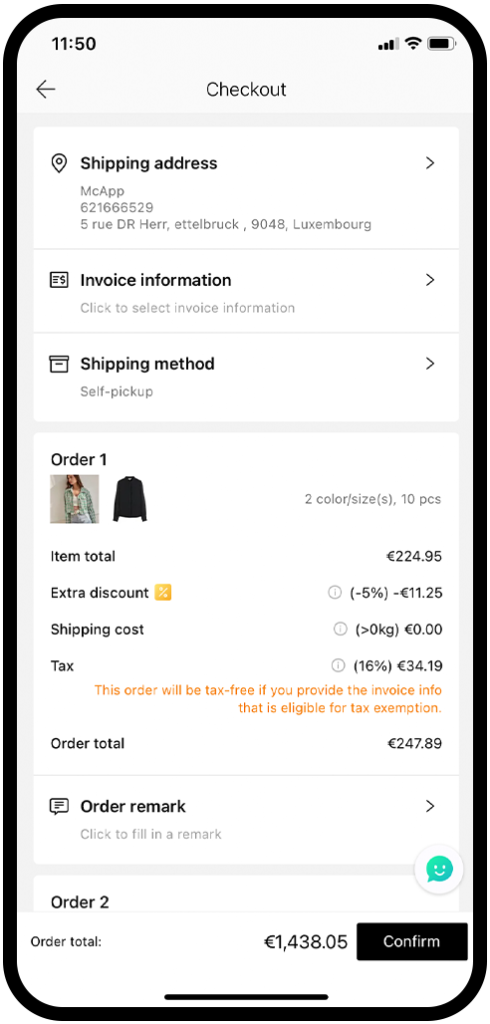A screenshot from a mobile phone displaying a detailed checkout page. The phone has a black, curved edge, but it doesn't appear photorealistic. The screen shows a white background with black text.

In the status bar at the top, the time reads 11:50 on the left. On the right, there are four bars of mobile signal, three bars of WiFi, and an almost full battery icon.

In the center of the screen, the word "Check Out" is displayed, with a black back arrow underneath it followed by "Shipping Address."

Below these headings, there are several sections:

1. **Shipping Address:** 
   - "Mac App, 621666529, 5RUDRHERR, Ethelbrook, 9048 Luxembourg" with a right arrow.

2. **Invoice Information:** 
   - "Click to select," followed by another right arrow.

3. **Shipping Method:** 
   - "Soft pick up," with a right arrow.

For **Order 1:**
   - There is an image of a woman wearing a green jacket and another image of a black jacket beside it. The order lists "Two collar sizes, 10 pieces" with an item total of 224.95 euros.
   - An extra discount of 5% is applied, reducing the total by 11.25 euros.
   - Shipping cost for more than 0 kilograms is listed as 0 euros.
   - Tax at 16% amounts to 34.19 euros.
   - A note in yellow states: "This order will be tax-free if you provide the invoice info that is eligible for tax exemption."
   - The order total for this section is 247.89 euros.

There is a section titled "Order Remark," with a prompt to "Click to fill in the remark," followed by a right arrow. Below this section, there’s a green circle with a smiling speech bubble icon.

For **Order 2:** 
   - Details are not visible as it requires scrolling down.

At the very bottom, the total amount for all orders is shown as 1438.05 euros. A black button on the right side with "Confirm" written in white concludes the screen.